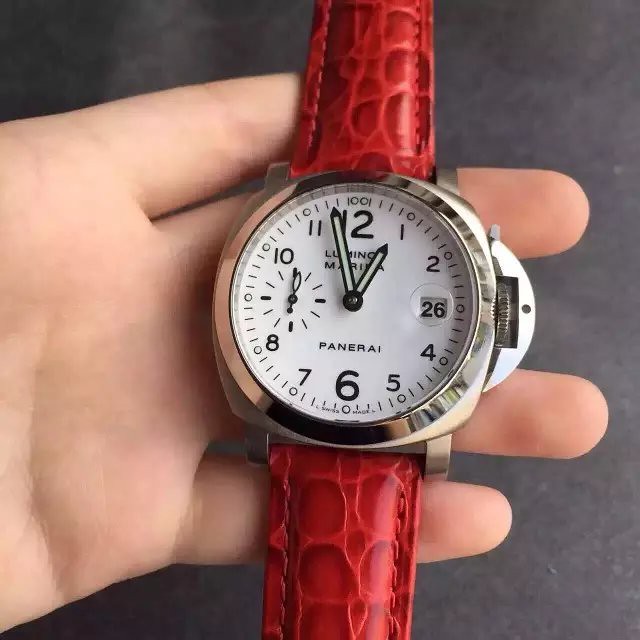In this close-up photograph, a light-skinned person's hand, splayed open, serves as a backdrop for a large wristwatch with a maroon red, crocodile-finish leather band. The watch, held palm-up against a dark gray table, features a silver housing and a white face accented with black borders and hashes. Prominent black Arabic numerals mark the hours, with larger numerals at 12 and 6. Numbers 3 and 9 are obscured by functional elements: the 3 by a small white square displaying the date '26' in black, and the 9 by a smaller sub-dial, likely indicating seconds, with a teardrop-shaped pointer. The hour and minute hands, outlined in black, have a faint fluorescent quality and are positioned just before 1:00 and almost reaching 12, respectively. An additional black-circled segment lies at the center of the face. Above the 6, the brand "Panerai" is inscribed in black letters. A crescent-moon-shaped guard protects the dial, adding to the watch's intricate detailing.